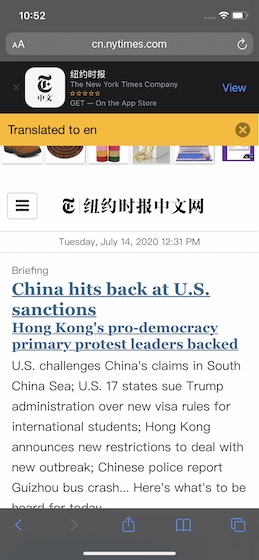A detailed screenshot from the New York Times website highlights several significant global news stories. At the very top, there is a partially visible interface element reading "translated to EN" with some Asian characters situated above the text "New York Times Company." Below, a section features content written in what appears to be Chinese. Further down, in English, the date and time are displayed as "Tuesday, July 14th, 2020, 12:31 p.m. briefing." The main headlines cover various international issues: "China hits back at US sanctions," "Hong Kong's pro-democracy primary protest leaders backed," "US challenges China's claims in the South China Sea," "US 17 states sue Trump administration over new visa rules for international students," "Hong Kong announces new restrictions to deal with new outbreak," and "Chinese police report Guizhou bus crash." At the very top of the image, the time "10:52" is shown alongside Wi-Fi and battery icons. The screenshot is oriented vertically, being taller than it is wide. The image contains no people, animals, birds, plants, flowers, trees, automobiles, or motorcycles.